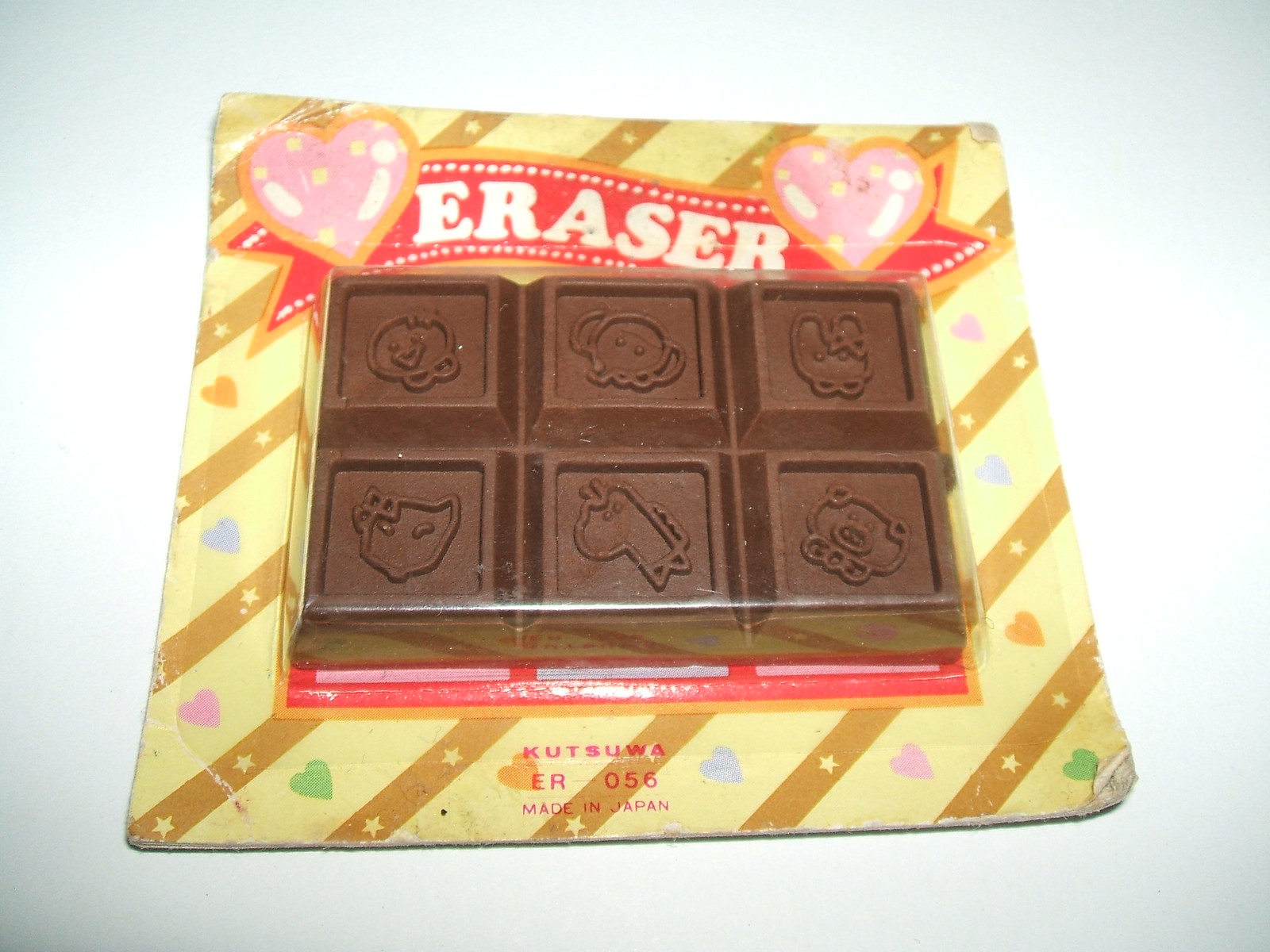The image depicts a brightly colored package resembling a chocolate bar, but upon closer inspection, it reveals that the contents are actually six erasers designed to look like pieces of chocolate. These erasers are connected in a block of six, arranged in three rows of two. Each eraser has a unique raised cartoon animal design on its surface, adding a playful touch. The packaging, detailed with yellow and gold stripes adorned with hearts in various colors (pink, orange, blue, and green), features prominent white lettering spelling "ERASER" on a red banner at the top, accompanied by two large pink hearts with white spots. The bottom of the package indicates that the erasers are made by Kutsuwa in Japan, with the text "K-U-T-S-U-W-A-E-R-056" visible. The background cardboard of the package shows signs of wear around the edges, and there is a noticeable glare from the plastic covering. This vibrant and eye-catching design is likely intended to appeal to children.